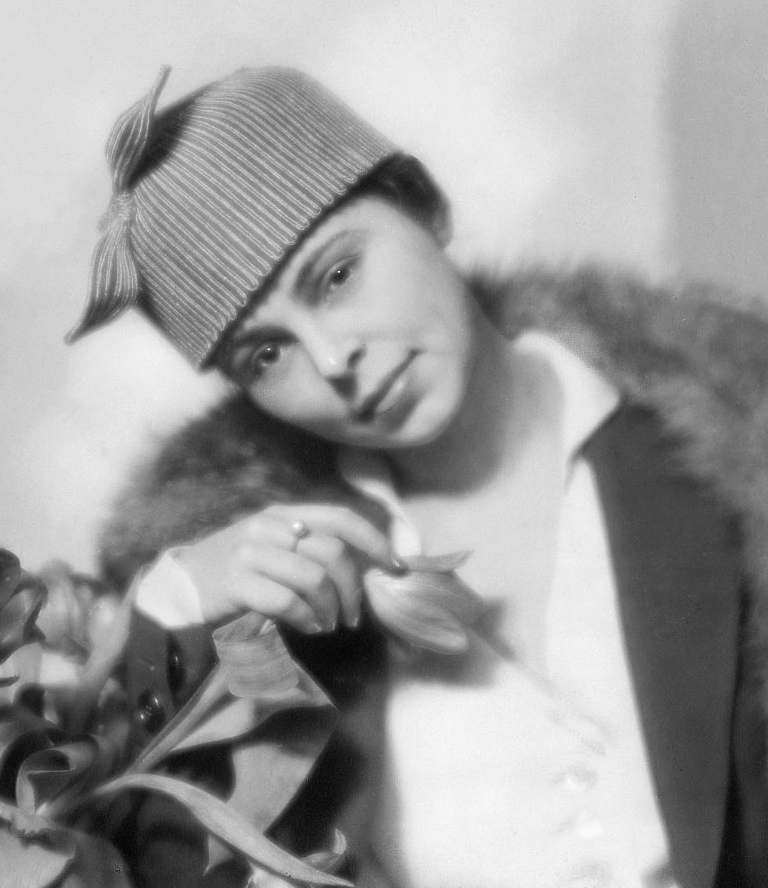This is an old black-and-white photograph, likely from the 1920s or early 1930s, depicting a young woman in her early 30s. She gazes directly at the camera with her head slightly tilted, wearing a wool cap adorned with a bow on top, covering her dark hair. The woman is dressed in a stylish coat with a fur-lined collar and a low-cut white blouse. Her right hand is visible, holding a tulip from a vase of flowers next to her, and she wears a distinctive ring on her middle finger. The background appears light-colored, and the photograph is square in shape.